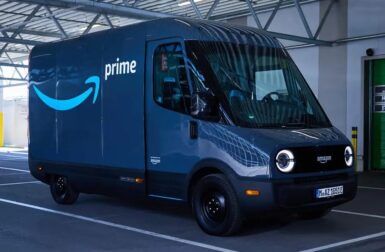The image features a large, dark blue Amazon Prime delivery truck parked indoors within a garage or warehouse. The truck, towering in stature, prominently displays the word "Prime" in white lettering alongside the iconic Amazon smile in a light blue hue on its side. The truck's sizable front windshield is visible, and the headlights appear to be illuminated. The surrounding area comprises neatly marked parking spaces that the truck occupies. The setting includes steel-framed ceilings and pristine white walls, contributing to the industrial ambiance of the space. Adjacent to the truck, a door is also visible, hinting at additional access points within this enclosed facility.